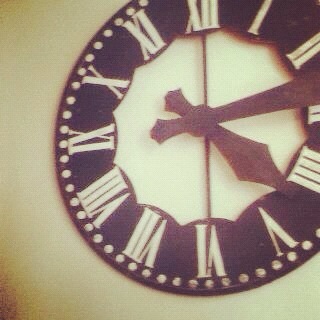This detailed photograph captures a black clock with a cut-out center, prominently positioned on a yellow wall that features a darker brown corner at the bottom left. The wall provides a stark contrast, bringing attention to the clock which occupies most of the top right side of the image. Adorning the clock's edge are white dots encircling it, adding a delicate border to its design. The clock face displays white Roman numerals starting with "XII" at the top, followed by a gap before "I," and continues with similar gaps between each numeral up to "XI," before repeating at "XII." The clock features two sword-shaped hands and a thinner, longer second hand which is positioned vertically. The minute hand is stationed between the Roman numerals "II" and "III," while the hour hand rests between "IV" and "V." The precise detailing of the numerals, hands, and surrounding dots contributes to its classic and elegant aesthetic.